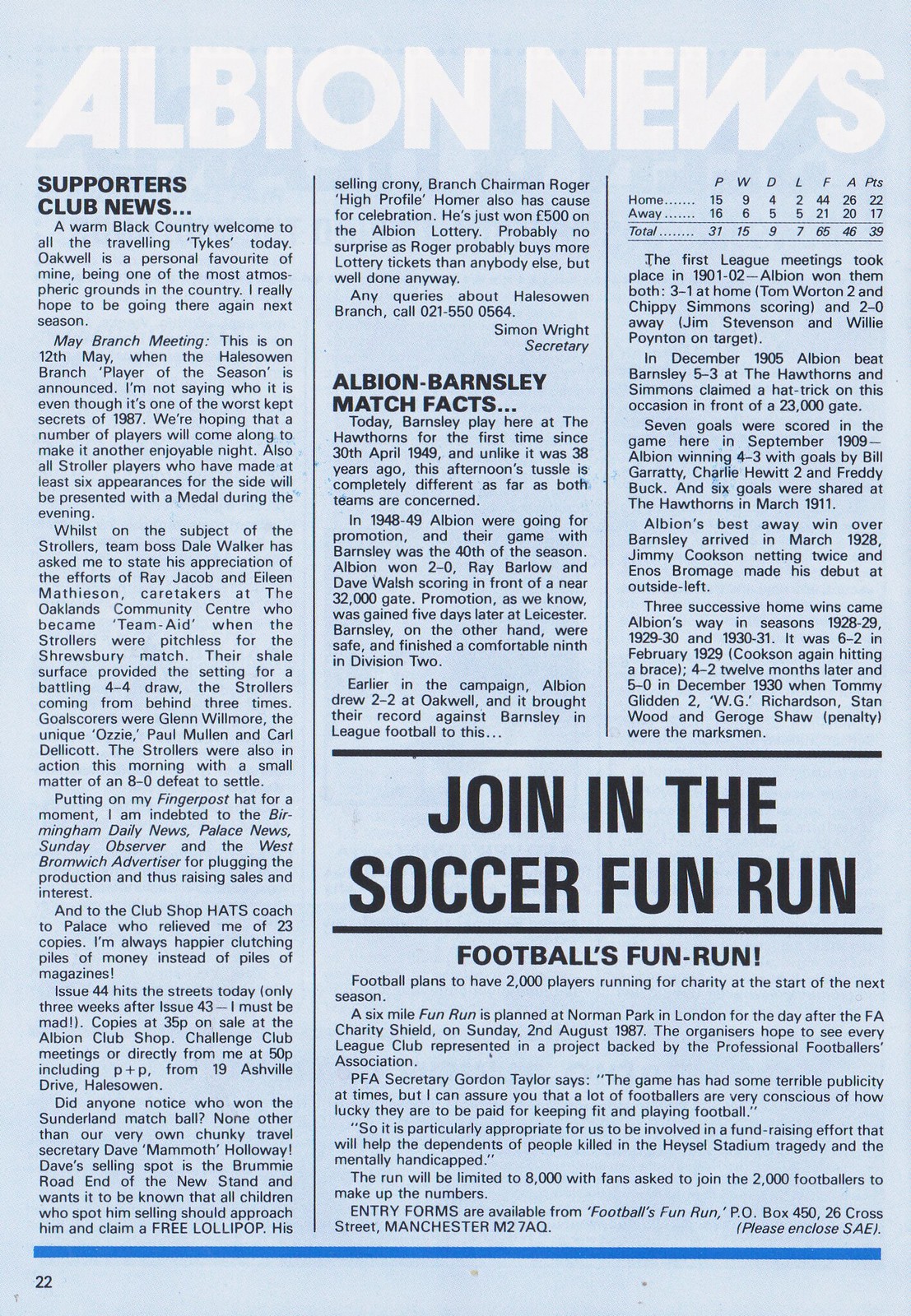The image depicts a detailed page from a magazine or newspaper named "Albion News," set against a light blue background with the title in bold white letters at the top. This page features various articles related to soccer, known as both football and soccer, with all text in black font. The page is divided into several columns, starting with "Supporter Club News" on the left, followed by "Albion Barnsley Match Facts," and a third section that appears to cover match statistics.

The Supporter Club News section warmly welcomes traveling tykes and highlights events such as the May branch meeting where the Player of the Season will be announced. It also recounts a dramatic 4-4 draw and an 8-0 defeat involving the Strollers, with a mention of key players and community figures. It humorously notes the publication success thanks to local media plugs, and even details how children can claim a free lollipop from a club member, Dave Mammoth, who sells in the new stand's Brummie Road End.

In the Albion Barnsley Match Facts section, it provides an extensive historical summary of past matches between Albion and Barnsley, featuring scores, notable players, and significant moments dating back to 1901.

Prominently displayed in a rectangular box towards the bottom right corner of the page, the headline "Join in the Soccer Fun Run" catches the eye, informing about an upcoming charity event for football fans and players alike. This event, planned for August 2, 1987, at Norman Park in London, encourages participation to support causes like the Hazel Stadium tragedy and mental health care. Additional information and entry forms for the run can be obtained from a Manchester P.O. Box, signifying strong community involvement.

The page concludes with a blue border, encapsulating a comprehensive view of recent happenings, historical insights, and community events related to Albion football.